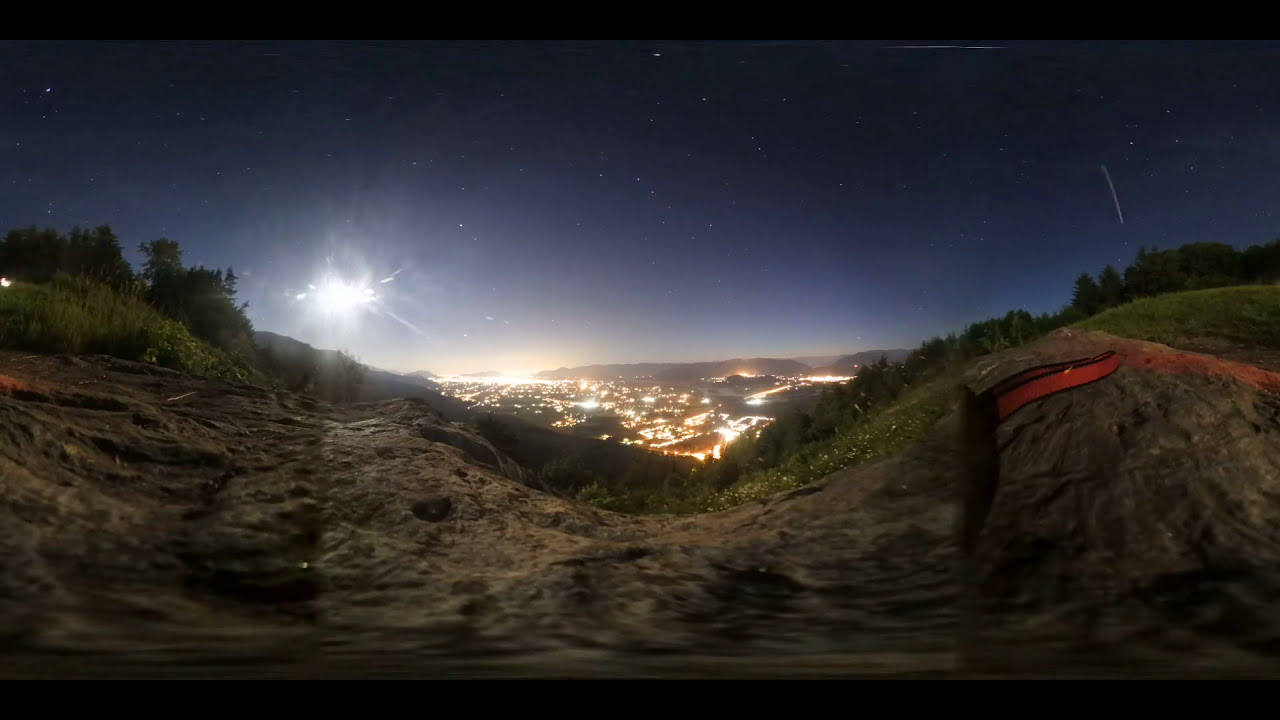The image depicts a scenic nighttime view from a high vantage point, likely a hill or mountain. In the foreground, there is a mix of rocky terrain and patches of green grass and bushes. As the terrain slopes downward, it transitions into a valley flanked by rows of lush green trees. Below, a sprawling city becomes visible, its multitude of lights illuminating the environment. Though the buildings aren't distinctly visible, the abundance of lights clearly marks the urban area. Beyond the city, a low mountain range extends across the horizon. The sky above transitions from a lighter blue, tinged with the residual glow of city lights, to a deeper, darker blue as night fully sets in. Stars begin to dot the sky, and a particularly bright, spiky light source on the left side of the image hints at either the moon or a strong artificial light, adding a dramatic touch to the celestial display.